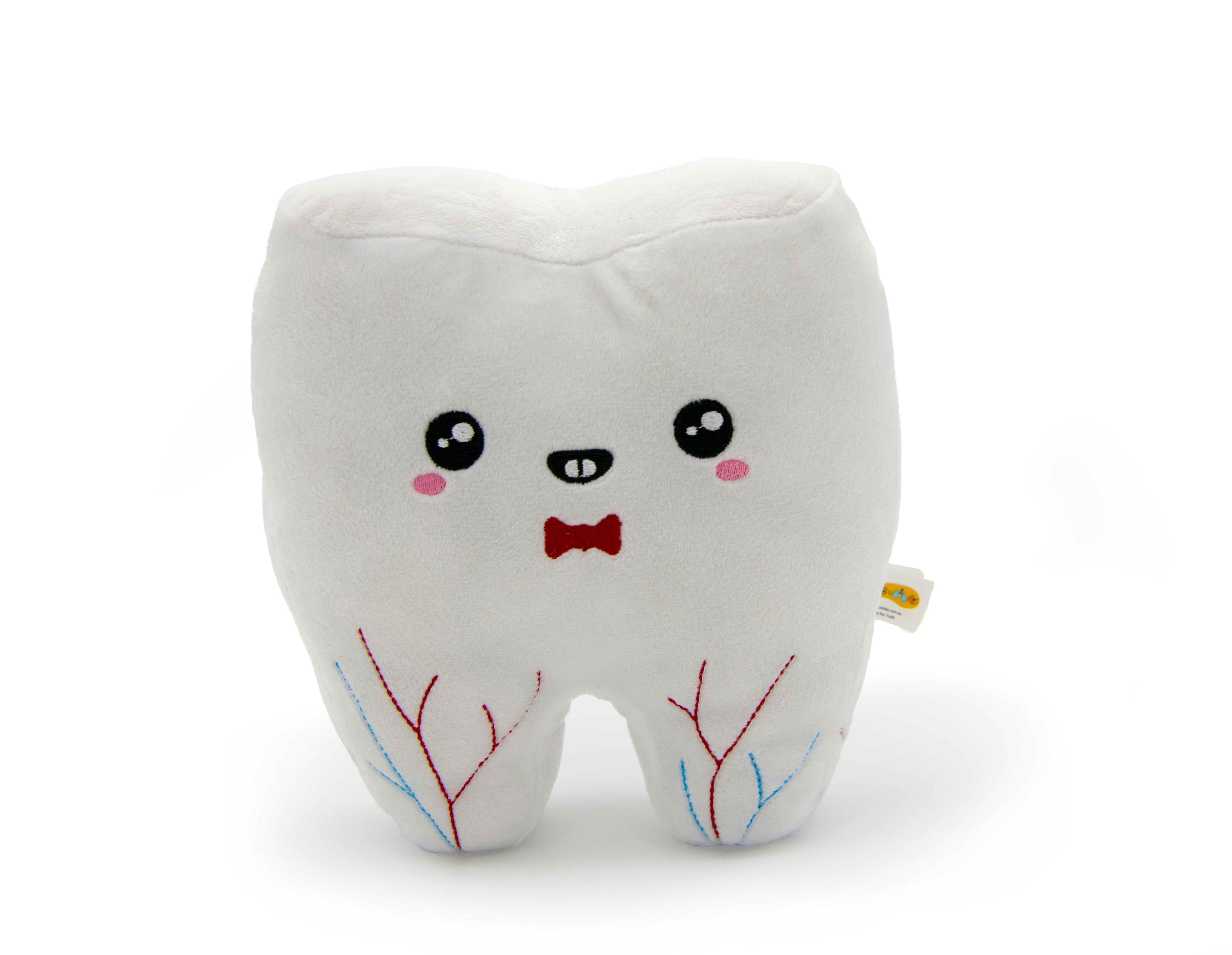This image features a cartoonish white pillow shaped like a human tooth, likely intended as a Tooth Fairy pillow. The plush toy has a whimsical design that includes a golden crown atop its "head." There are blue and red lines on each of the two roots extending from the bottom, representing veins or arteries. The tooth character has two cute black eyes with white specular highlights, a small triangular black nose with white dots, and a wide, cheerful red mouth adorned with a small red bow tie beneath it. Blushing pink circles on its cheeks add to its charming appearance. A tag is attached to the right side of the plush toy, though its details are not legible. The material seems synthetic and velvety, suggesting it may be fuzzy or made from velour. The photo appears to have been taken casually with a phone rather than professionally.